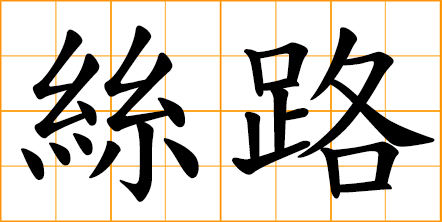This image showcases two Chinese ideograms, set side by side against a background of a thin orange grid composed of 16 smaller squares, arranged 4 across and 4 down. Each ideogram occupies its own grid space with a thin orange border. Both ideograms are rendered in black with computer-generated precision, featuring predominantly angular and swooping lines. The ideogram on the left resembles two sideways W shapes or V shapes stacked on top of each other, with three dot-like teardrops underneath the first W. From the second W, a tree branch-like structure extends outward, adorned with teardrops. The ideogram on the right includes a square with vertical and horizontal lines extending from it, followed by a prominent X-pattern and another square beneath it. Both ideograms emphasize distinct geometric and flowing elements, intricately arranged to form their unique structures.